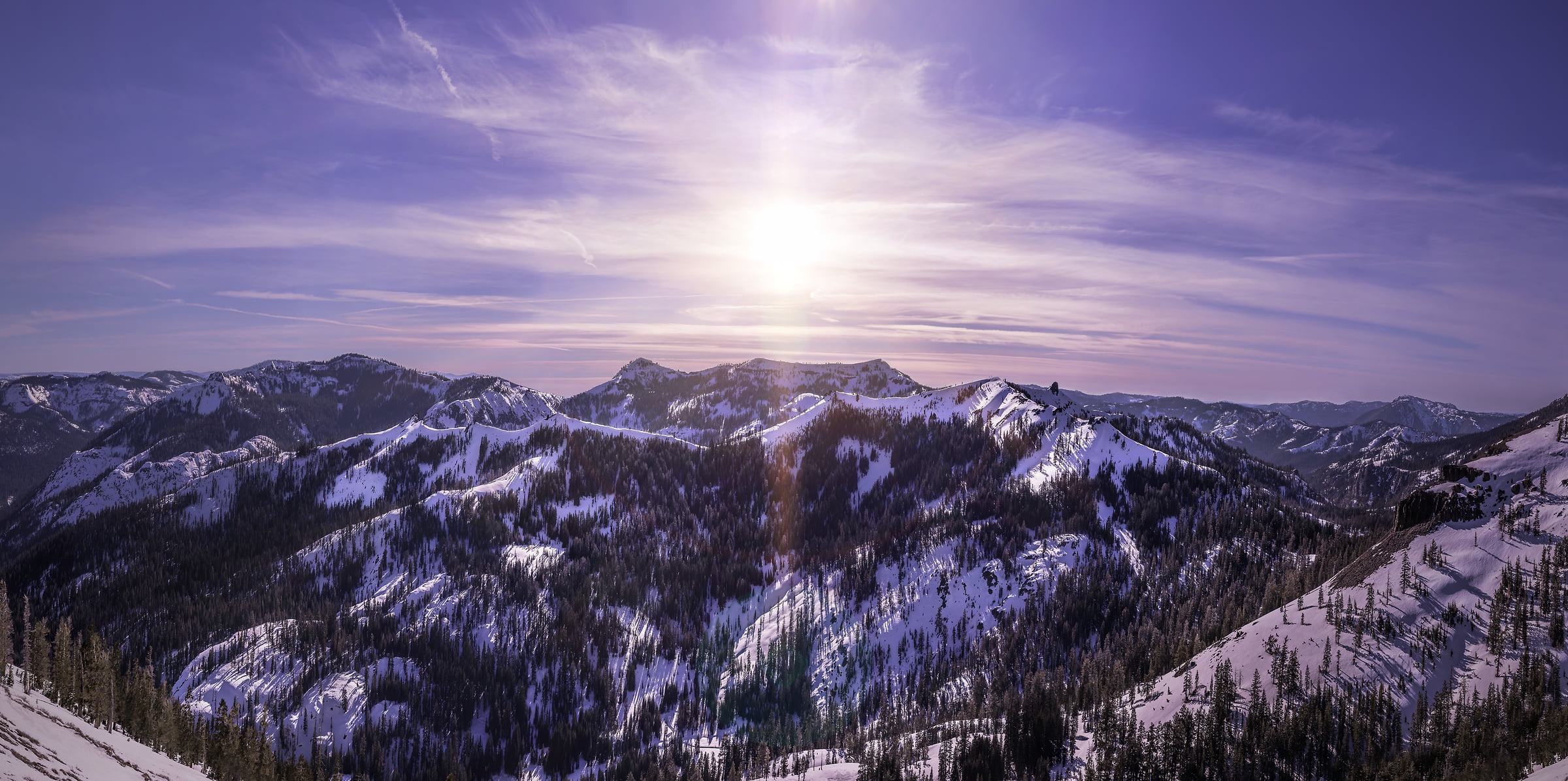In this photograph, the viewer is presented with a breathtaking winter mountain landscape. The scene showcases a continuous range of snow-capped mountains, their peaks uniformly rising and falling in a horizontal sweep across the image. The ground is blanketed in thick snow, dotted with numerous dark green, pine-like trees resembling Christmas trees. These trees, while sparse and scattered, contribute to the alpine beauty of the scene.

Dominating the upper half of the photo is a crisp, light blue sky that almost verges on a purple hue, adorned with wispy, sheer, vapor-like clouds that streak across the horizon. At the very center of the sky, a bright, white light—likely the sun—bursts through the thin clouds, casting rays in all directions and creating a luminous focus that highlights the serene wintry setting below. The sun's position and the quality of light suggest a winter day, with no visible man-made structures to interrupt the natural splendor.

In the bottom left of the photograph, a ridge lightly dusted with snow provides a lead-in to the more prominent central mountains, whose gray rocky faces peek through their snowy coverings. The visual composition of the photograph is balanced, offering a slight dip at either end of the horizon, giving a subtle sense of depth and grandeur to the mountain range. The overall mood of the image is tranquil and pristine, capturing the raw, untouched beauty of this high-altitude, alpine environment.